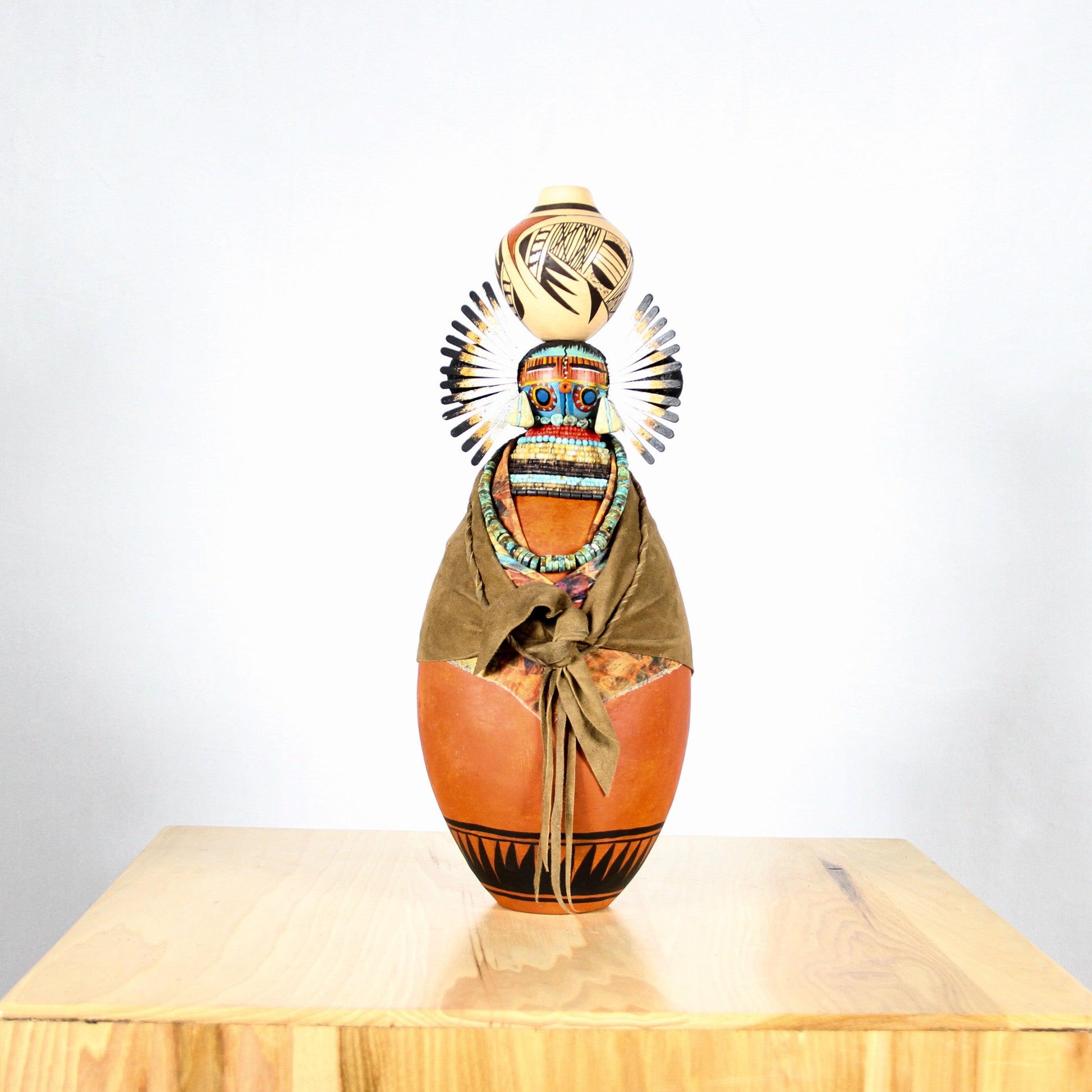An intricately designed Native American vase sits prominently on a square, thick piece of light-colored wood, set against a white wall. The vase itself is a striking orange hue, adorned with black circles at the bottom from which black lines ascend. A dark brown cloth is wrapped around the middle, tied together neatly, and serves as the base for an elaborate necklace featuring beads of light and dark turquoise, black, and brown. The upper part of the vase is designed to resemble a face, with two blue circles for eyes and a light brown section with black lines above the eyes. 

Above the face-like section, the vase narrows like a neck, displaying a series of colorful lines: black, light blue, more black, yellow, and a teal stripe. At the very top, the vase supports a small yellow ceramic bowl, which is adorned with intricate green and orange designs and slopes upward to a circular opening. Surrounding this bowl, metal pieces resembling sun rays extend outward, with gray tubes on the right side and black tubes on the left. Subtle details like beads and paint intensify the facial features, while elements resembling earrings and a feathered headdress accentuate the sides of the head. A white light shines from behind, enhancing the vase's vibrant colors and detailed craftsmanship.